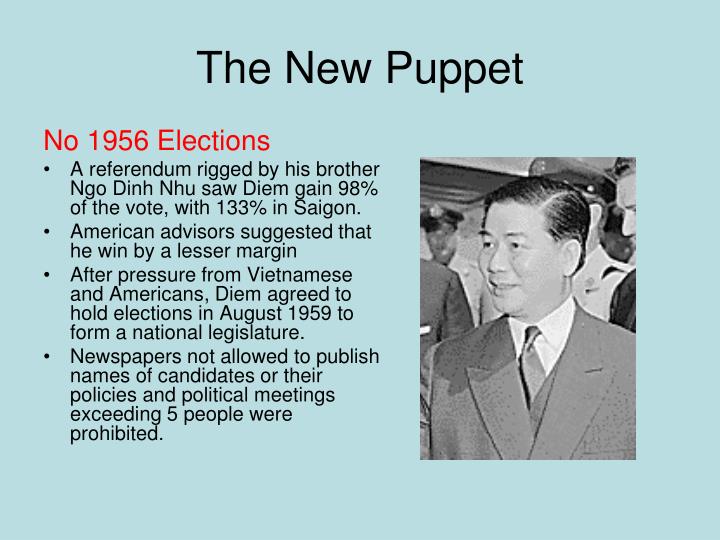The image is a digitally synthesized content slide from a presentation. It features a light blue background with the title "The New Puppet" in large black text at the top center. On the left side, there is a red text caption that reads "No 1956 Elections" followed by a series of four bullet points in smaller black text. The bullet points state: 

- A referendum rigged by his brother Ngo Dinh Nhu saw Diệm gain 98% of the vote with 133% in Saigon. 
- American advisers suggested that he win by a lesser margin. 
- After pressure from Vietnamese and Americans, Diệm agreed to hold elections in August 1959 to form a national legislature. 
- Newspapers were not allowed to publish names of candidates or their policies, and political meetings exceeding five people were prohibited.

On the right side of the image is a black-and-white photograph of an Asian man with dark hair, wearing a dark suit. He is the focus of the image, and behind him, there are several people, possibly officials, who appear to be wearing caps. The man in the photograph is looking off to the left.